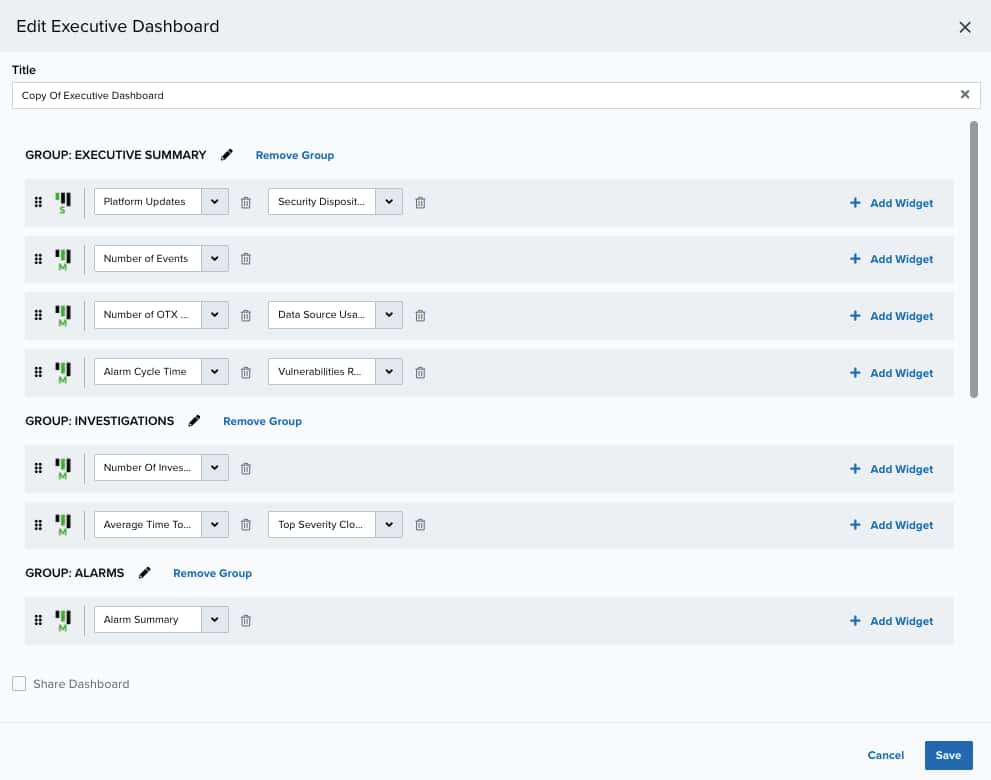This image captures a detailed view of a web page or application interface focused on automation and processing, presented in portrait orientation. The background is not distinctly defined, and the image is slightly taller than it is wide. 

At the top of the interface, there is a grey bar with black text displaying "Edit," "Executive," "Dashboard," and an "X" in the right corner, presumably to close the window. Below this, a lighter grey box features the word "Title" in small black text, followed by a larger box with the text "Copy of Executive Dashboard" also in black font, with another "X" for closing.

Following this section, a black header reads "Group Executive Summary" accompanied by a pencil icon indicating an option to edit, alongside a blue "Remove Group" button. 

Beneath this, there is a cluster of four individual grey boxes labeled "Platform Up," each containing dropdown menus. The dropdown options include:
- "Platform Updates" and "Security Disposition"
- "Number of Events"
- "Number of OTX" and "Data Source"
- "Alarm Cycle Time" and "Vulnerabilities"

Each box has a blue "Add Widget" button to the right.

The subsequent section, titled "Group Investigations," consists of two grey boxes with the following headers and options:
- "Number of Investments"
- "Average Time" and "Top Severity"

This section also includes the "Add Widget" option and the "Remove Group" button for each header.

The last section, labeled "Group Alarms," features a grey box with the header "Alarm Summary," along with the same "Add Widget" and "Remove Group" options.

At the bottom right corner of the interface, there are two buttons: a blue "Cancel" button and a "Save" button with a blue border and white text. These buttons provide options to either cancel the current actions or save any changes made to the dashboard settings.